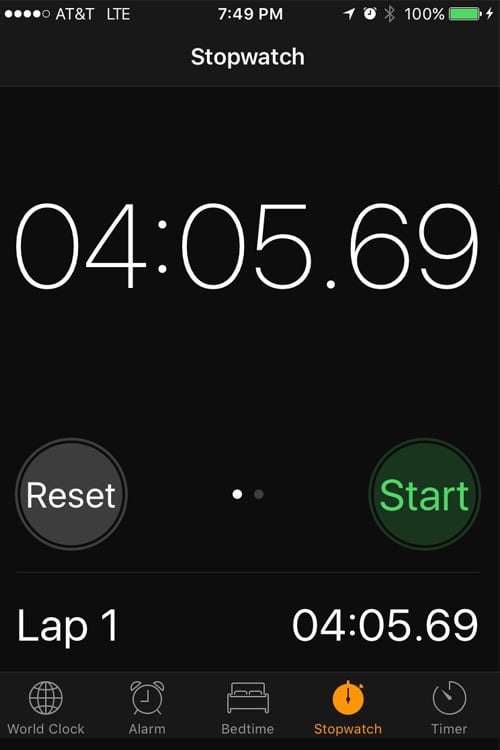Caption: 

A detailed view of an iPhone stopwatch. The screen features a sleek black background with white text. At the top, the status bar displays the AT&T network with full LTE signal strength, and a green battery icon indicating the phone's charge level. The current time is shown as 7:49 PM. Below the status bar, the stopwatch interface displays a running time of 4 hours, 5 seconds, and 69 hundredths of a second. 

There are two prominent buttons underneath the time: a black "Reset" button on the left and a green "Start" button on the right. The lap time is noted as "Lap 1" with the same time of 4:05:69. At the bottom of the screen, five icons are visible, representing the different functionalities of the clock app: World Clock, Alarm, Bedtime, Stopwatch, and Timer. The Stopwatch icon is highlighted in orange, indicating the current active mode. 

The overall layout features predominantly black and white colors, following Apple's design aesthetics, which are distinct from other brands like Samsung Galaxy.